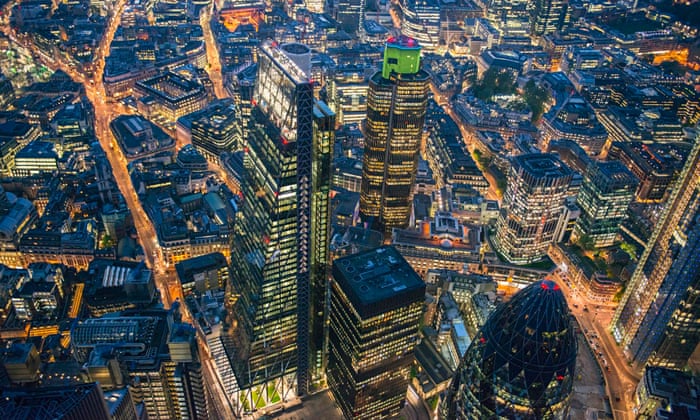An aerial view of a bustling metropolitan area showcases a labyrinth of irregularly shaped blocks teeming with life. Dominating the center are three skyscrapers closely clustered together. The tallest, on the left, features a pyramid-like structure that widens at the base and narrows at the top, consisting of 25 to 30 floors. To its right stands a shorter, rounded building adorned with a green drum-like structure on the rooftop, possibly a water tank, along with airplane morning lights. The third, slightly smaller, skyscraper completes the trio. The cityscape is characterized by predominantly dark buildings, which appear black or dark blue from above, but their surfaces are intermittently illuminated by the yellow glow from countless windows. The streets below are painted in a golden-yellow hue, reflecting the headlights of the numerous cars traversing the roadways. Despite the tight and cluttered appearance of the city, the overall scene exudes a vibrant and dynamic urban pulse, with every inch of the image filled with buildings and traffic.